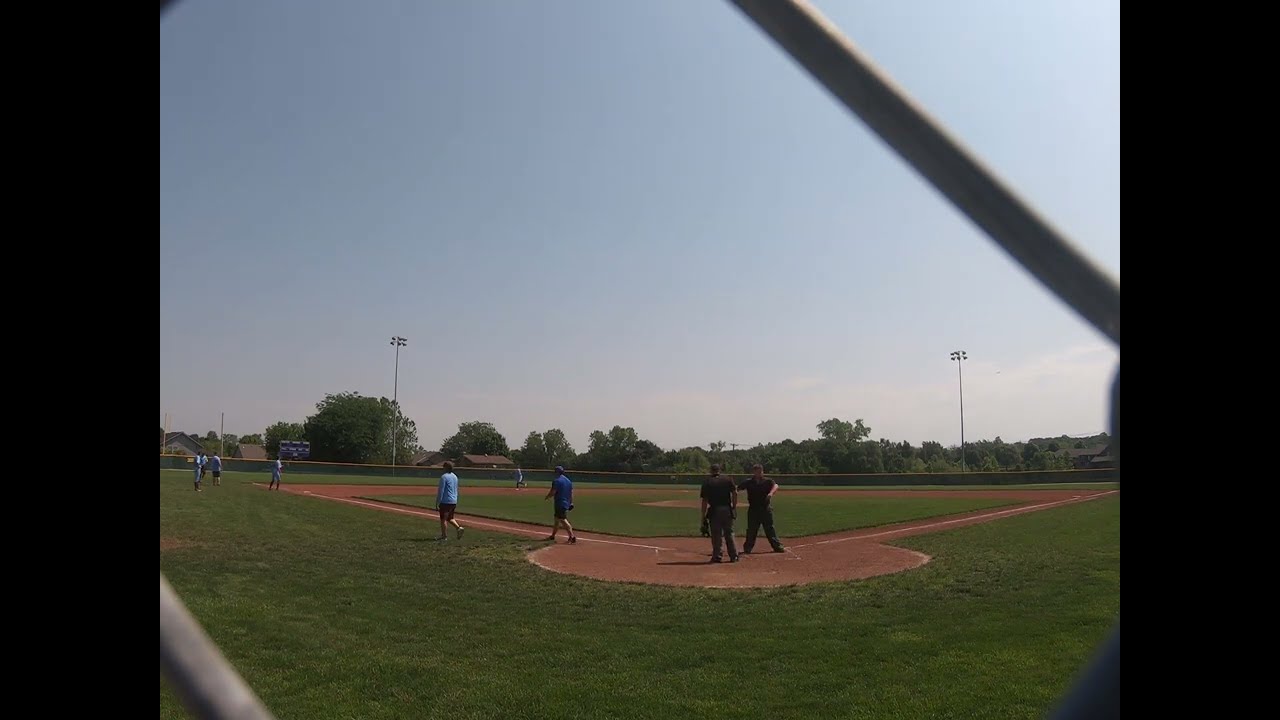The image depicts a vibrant baseball game from the viewpoint of someone standing behind the batter's cage. At the center of the image is a well-maintained baseball diamond with vivid green short grass contrasting the brown dirt areas marked with crisp white chalk lines. Two umpires, identifiable by their black polo shirts, black pants, and black caps, stand prominently next to home plate. One umpire is holding protective gear, and both are facing towards the pitcher's mound. To their left, there are several players dressed in light blue shirts and shorts, likely on the third baseline, with one person positioned out in the outfield. Surrounding the field, a green fence is visible with houses peeking over it, and tall lights tower over the background, though currently unlit as it is midday. The sky forms the upper half of the composition, while the field occupies the lower half, completing this picturesque daytime scene at what appears to be a little league or high school baseball field.